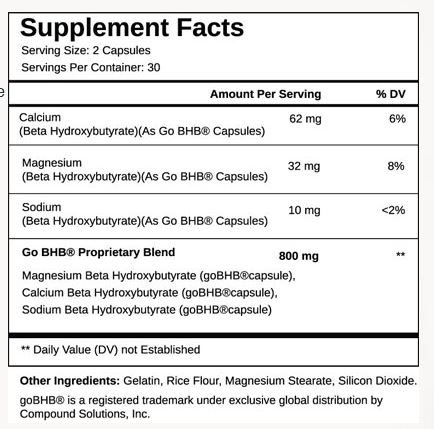This image features a Supplemental Facts label, common on over-the-counter pharmacy supplements, against a very light gray background that subtly contrasts with the white label itself. The label is framed with a thin black line, adding definition to the box. At the top in bold black letters, it reads "Supplemental Facts," followed by key information: "Serving size: two capsules," "Servings per container: 30." A thicker black line separates this section from the nutrient details below. 

The main section lists the amounts per serving and their corresponding % Daily Value (DV) in bold text. It includes:
- Calcium: 62 mg (6% DV)
- Magnesium: 32 mg (8% DV)
- Sodium: 10 mg (less than 2% DV)
- GoBHB (a proprietary blend): 800 mg

At the bottom, within the square, it includes secondary information such as "Magnesium beta-hydroxybutyrate" and an asterisk noting that the daily value (DV) is not established for some ingredients. Below this, outside the outlined box, additional ingredients are listed: gelatin, rice flour, magnesium stearate, silicon dioxide.

This detailed Supplement Facts label provides a clear and standard presentation of the supplement's nutritional content and additional components, all set against a distinguishable light gray backdrop.